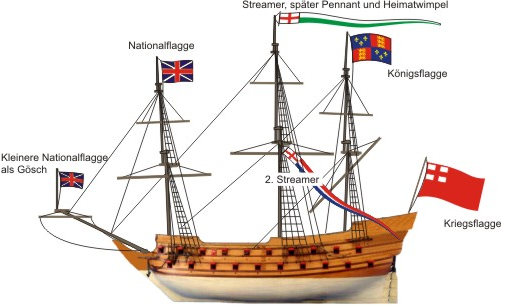The image depicts a detailed model of an old wooden sailing ship against a pure white background. The ship, viewed from the side, faces left and features a rich brown upper deck with a lighter brown or milky bottom. It has a curved base with a central spine and is adorned with two rows of holes along its side. Multiple masts extend from the top of the ship, from which various flags and streamers are attached. Prominently, a streamer features the inscription "Krieg's flag," with "K-R-I-E-G-S-F-L-A-G-G-E" spelled out. Another flag displays a red cross and a white and red design. These flags, along with a banner labeled "Nationalflagge" (a German term for national flag), highlight the ship's adorned and historic aesthetic. The masts are equipped with ropes, adding to the intricate details of this maritime model.